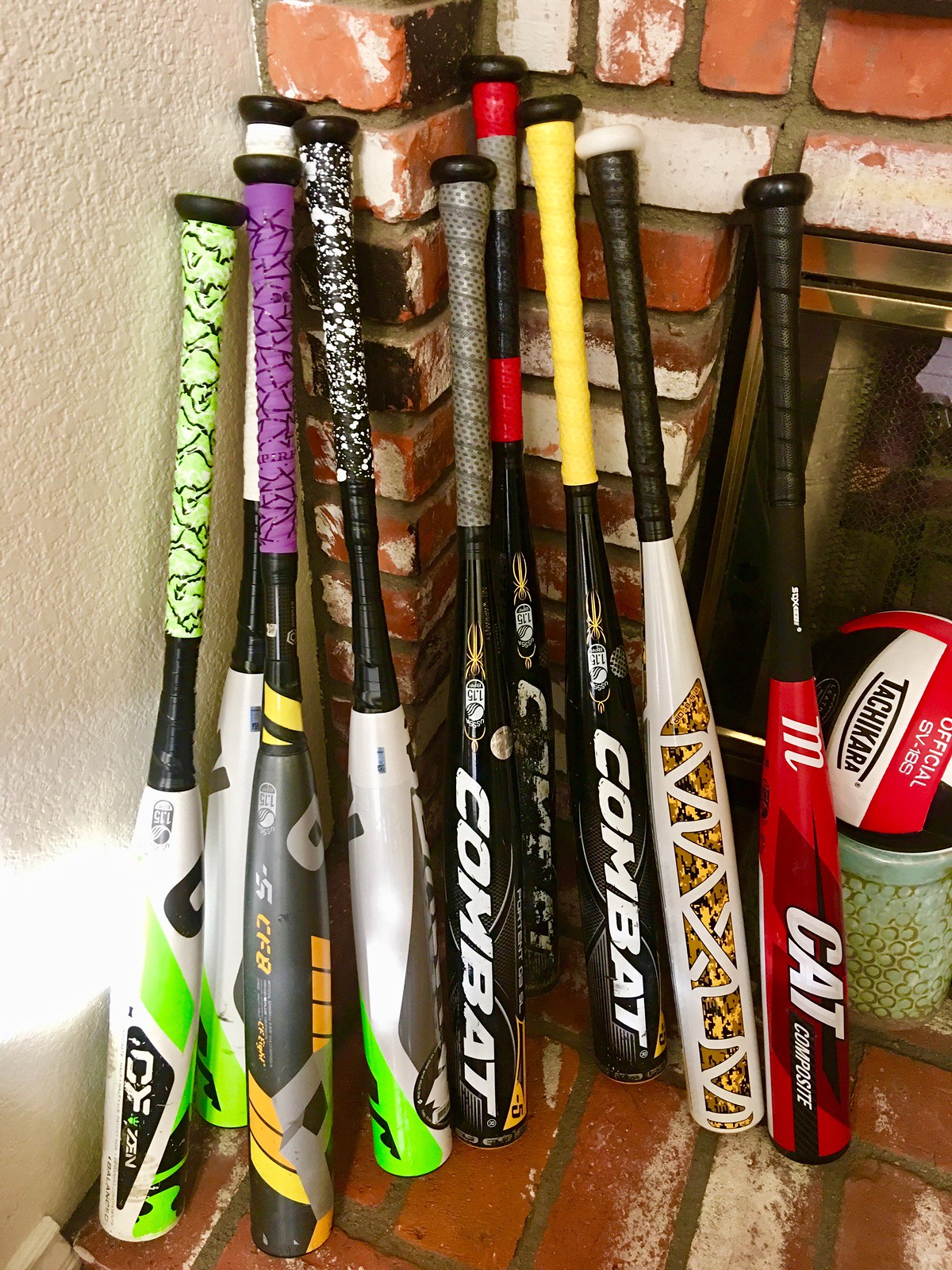The photograph, captured with a high-quality camera for clarity, prominently features a collection of nine metal baseball bats or softball bats arranged in front of a traditional red brick fireplace with a gold fire fence. These aluminum bats, each standing with their handles facing upwards, showcase a range of colors and grip tapes. The bats include hues such as white, black, silver, green, bright yellow, light green with black stripes, purple with black stripes, and a distinctive black and white pattern. They also feature various brands, including Combat and Cat. Adjacent to the bats, there's a small red, white, and black ball. The left wall, visible in the background, is beige with a textured finish, complementing the homely indoor setting. The green ceramic bucket positioned near the fireplace contributes an additional detail to this meticulously captured scene, potentially intended for selling items online.